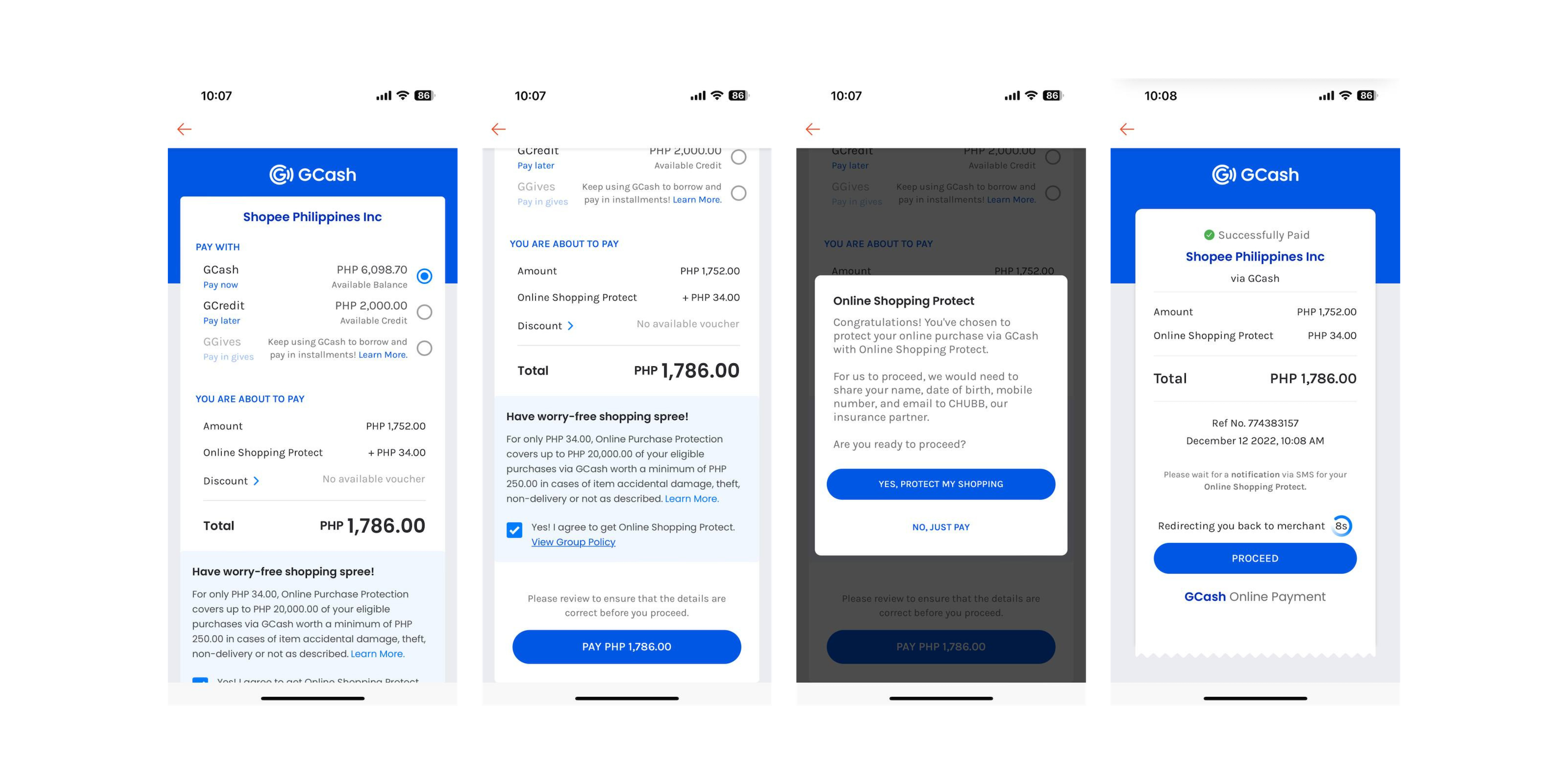The edited image showcases four phone screens aligned horizontally, each featuring different aspects of the Gcash app. On the far left of the image, there's the logo for Shops Philippines Inc., followed by the text "Pay with" and three selectable payment options, with Gcash highlighted. The first screen displays the Gcash payment page detailing the amount to be paid, including the order cost, shipping fee, and the total amount at the bottom. Small blue text indicates "You are about to pay."

The second screen highlights the bottom section of the payment page, showing the total price. Below, a checked blue box displays the option “Move worry-free shipping spree” with a "Pay" button prominently featured at the bottom.

The third screen captures a pop-up titled "Online Shopping Protect," which appears when the corresponding option is selected. The message includes “Yes, protect my stuff” in blue, signifying a confirmation choice.

The fourth and final screen revisits the payment confirmation for Shops Philippines Inc. via Gcash, detailing the amount, online shipping, total, and displaying the current date and time. A "Proceed" button in blue is visible at the bottom, indicating the final step to complete the transaction.